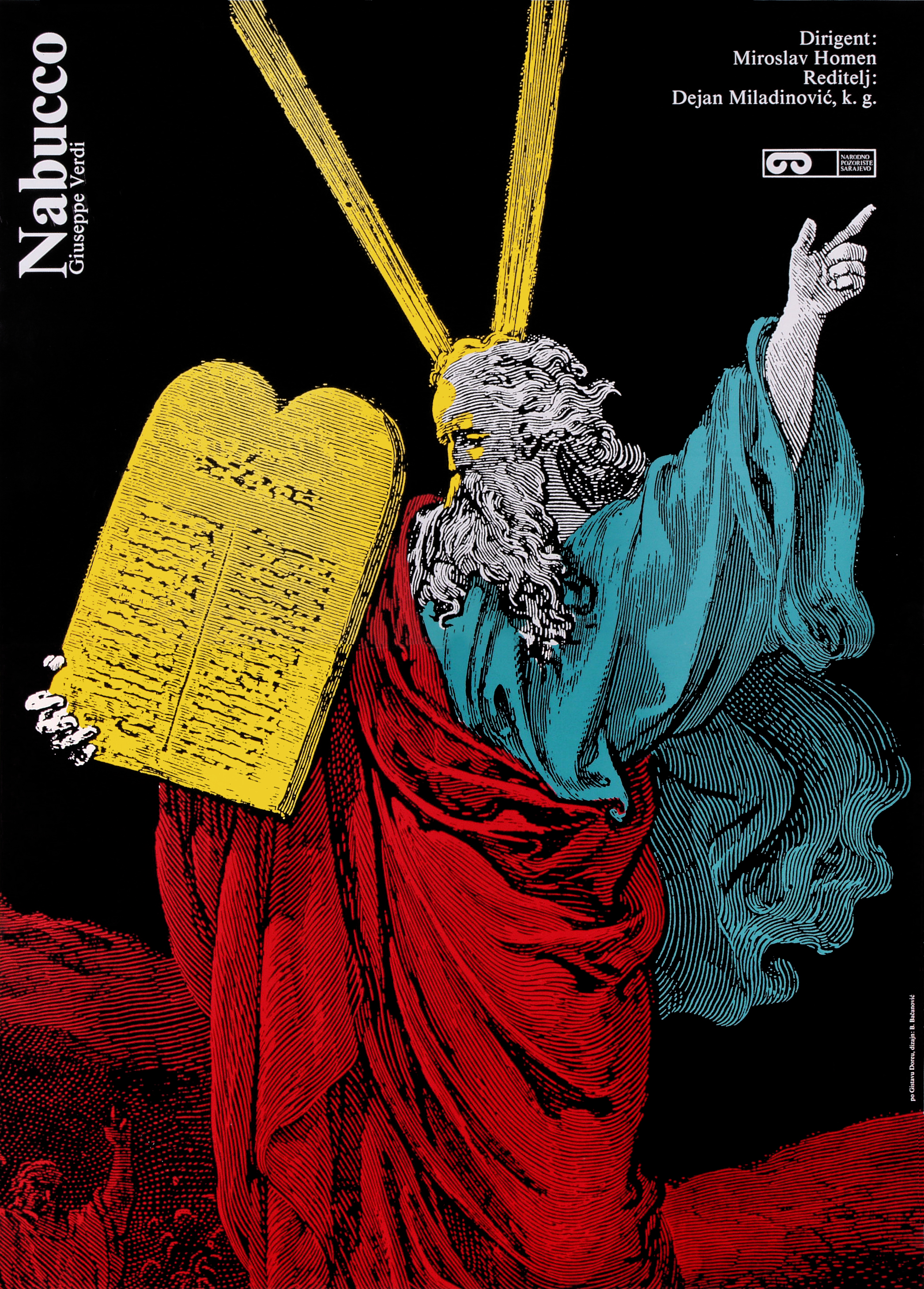The digital artwork depicts a biblical scene of an older man, likely Moses, holding up a yellow stone tablet believed to be the Ten Commandments. Moses is adorned in period clothing: a red robe draped over his left shoulder and a teal robe beneath it, flowing down to the bottom of the painting. He has long white hair and a long white beard, with his left hand pointed towards the sky, signifying a divine connection. Two broad beams of light emanate from his head in a V-shape, further emphasizing his holy stature. The background is stark black, providing contrast to Moses' vibrant attire and the red hue that seems to envelop the ground and the people below, who appear to be in joyous exaltation. Text on the image reads, "Nabucco Giuseppe Verdi Dirigent Miroslav Homan Radisic Dejan Miladinovic KG," with possible reference to a performance or recording, indicated by a Dolby Sound logo in the corner.